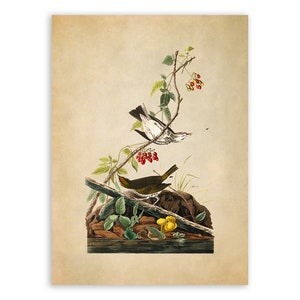The image captures a detailed, Japanese-inspired artwork presented on a slightly worn, beige paper with a thick tan border. The centerpiece features a realistic painting of nature with elements meticulously placed throughout. In the middle of the composition, there is a small patch of brown soil and black rocks, punctuated by a diminutive green plant. An angular brown stick extends through this terrain, hosting a pair of dark brown birds. One bird perches atop the stick, while another finds footing on a small tree emerging from the ground, adorned with green leaves and red berries. More green leaves and clusters of red berries populate the upper sections of the tree. Additionally, a yellow fruit or flower can be spotted at the base of the stick. The overall scene, though confined within the small canvas, evocatively captures a rich slice of natural life, rendered in a style that hints at eastern artistic traditions.